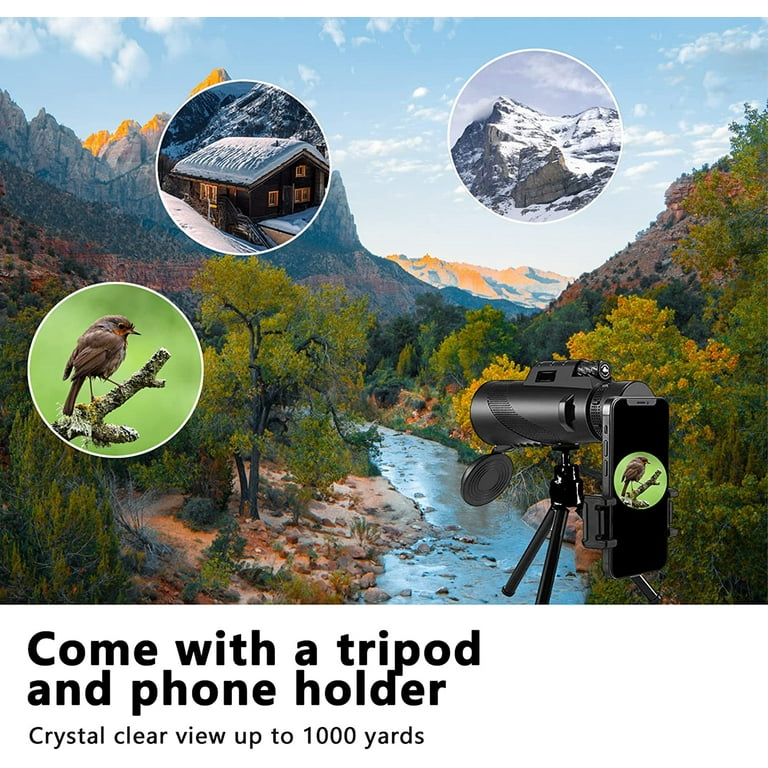This image, seemingly an advertisement, features a breathtaking outdoor landscape. Predominantly showcasing a mountain valley scene, it presents lush trees and towering peaks on both sides, with additional snowy mountains visible in the distance under a blue sky dotted with white clouds. A river meanders through the valley floor, enhancing the natural beauty of the scene. In the bottom right-hand corner, there is a black tripod set up, supporting a camera attached to a smartphone. The phone screen displays a photo of a brown bird perched on a twig. This image is simultaneously magnified and superimposed in a white-outlined circle on the main photograph. Adjacent to it, two more white circles display detailed images: one of a snow-covered log cabin and another of a snowy mountain peak. Below the main image, black text reads: "Comes with a tripod and phone holder, crystal-clear view up to 1,000 yards."